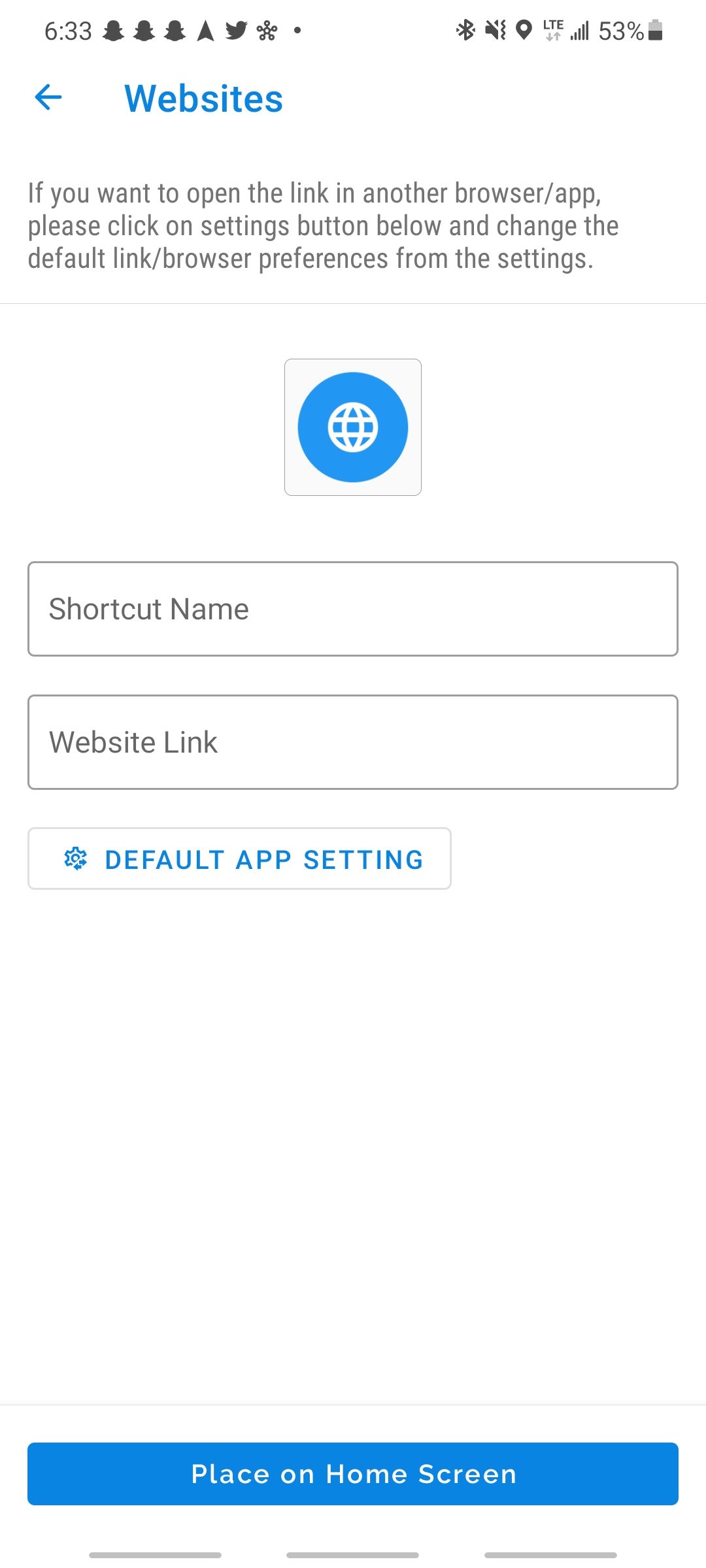This is a screenshot of a mobile device's screen. At the top, the status bar displays the time as 6:33, along with a series of notification icons including three Snapchat icons, a Twitter icon, a Bluetooth icon, a stylus icon, and an LTE signal indicator. The battery level shows 53% remaining. 

Below the status bar, there is a section with the word "WEBSITES" prominently displayed in bold, blue letters. The paragraph that follows advises users that to open links in another browser app, they should go into the settings and change the default link browser preferences. 

The interface includes a blue circular icon featuring a small globe, and a square icon outlined in grey. Additionally, there are two white input boxes labeled "Shortcut Name" and "Website Link." A blue button labeled "DEFAULT APP SETTINGS" in all caps is present, with another blue button below it reading "Place on Home Screen" in white text.